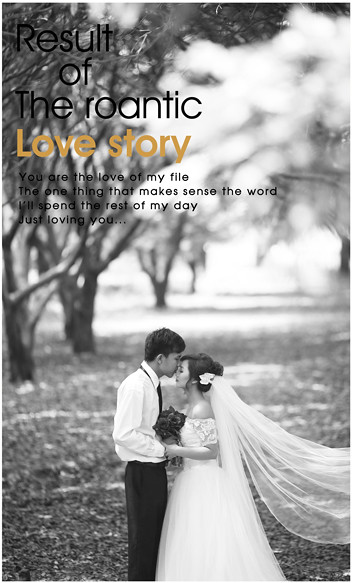The black and white promotional image depicts a heterosexual couple on their wedding day, set outdoors in a tree-lined area. A pathway covered in leaves stretches through the center of the image, emphasizing the natural, romantic setting. The couple, positioned at the bottom of the vertical image, leans into a tender kiss. The bride, dressed in a strapless white wedding dress with a flowing veil, is holding a bouquet as she faces her groom. The groom is angled towards her, seemingly kissing her on the forehead.

Overlaying the image, though difficult to read due to the black text blending with the background, is a heartfelt message in the top left corner. It reads: "Result of the romantic love story. You are the love of my life, the one thing that makes sense, the word. I'll spend the rest of my days just loving you." This emotional text, despite some typographical errors, reinforces the image's theme of enduring love.